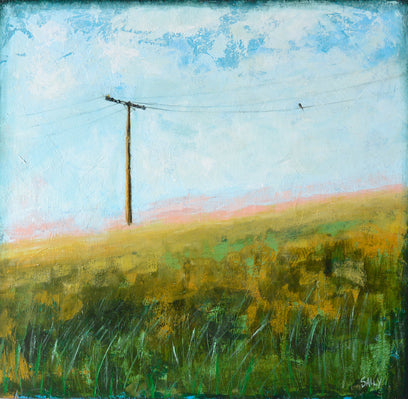This painting, presented on a small, square canvas, depicts a serene rural scene dominated by a field and a towering telephone pole. The field stretches across the bottom of the painting, featuring dense green grass interspersed with patches of yellow that might represent flowers. Above the field, the sky showcases a blend of light blue hues and white, wispy clouds that partially obscure a clear blue expanse behind them. A single bird can be seen perched on the wire extending from the wooden telephone pole, which stands prominently at the center of the composition. The pole has a single crossbar with several wires fanning out, adding a touch of structural detail to the tranquil landscape. Hints of pink along the horizon add depth to the sky. The painting's style is slightly blurred, evoking a soft, almost dreamy atmosphere. The primary colors in this artwork include green, yellow, various shades of blue, white, brown, and black, with no text visible within the image. This professionally crafted piece captures a peaceful moment in the countryside, with meticulous attention to the interplay of color and form.